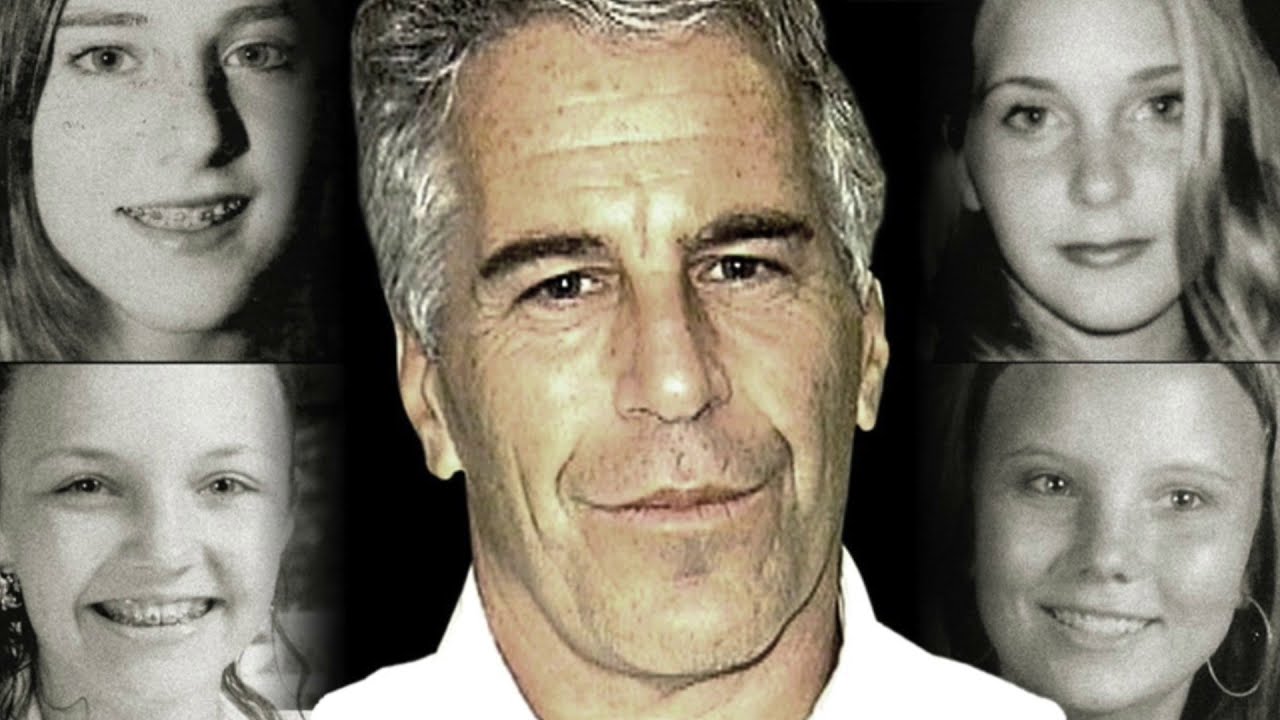The image is a close-up headshot of Jeffrey Epstein, likely taken from a news story or a newspaper. Epstein, an older Caucasian man with peppered gray hair and a large forehead, is looking directly at the camera. His hair is slightly cropped at the top, and he has dark eyebrows, visible forehead lines, and wrinkles on his cheeks and under his eyes. He sports a bit of facial stubble and is wearing a white collared shirt. Surrounding Epstein's image are four monochrome photographs of young girls' heads. 

In the top left is a girl with freckles and braces, smiling; she appears to be between 12 and 14 years old. Below her, another girl with wavy hair pulled back, also with braces, looks slightly younger or the same age. On the top right, a girl with long blonde hair has a closed mouth, and on the bottom right, another blonde girl with a visible hoop earring on her left ear is smiling. These girls also seem to be around 12 to 14 years old. All the girls look white, and their images are positioned around Epstein's headshot, creating a stark contrast between the central adult figure and the surrounding youthful faces.